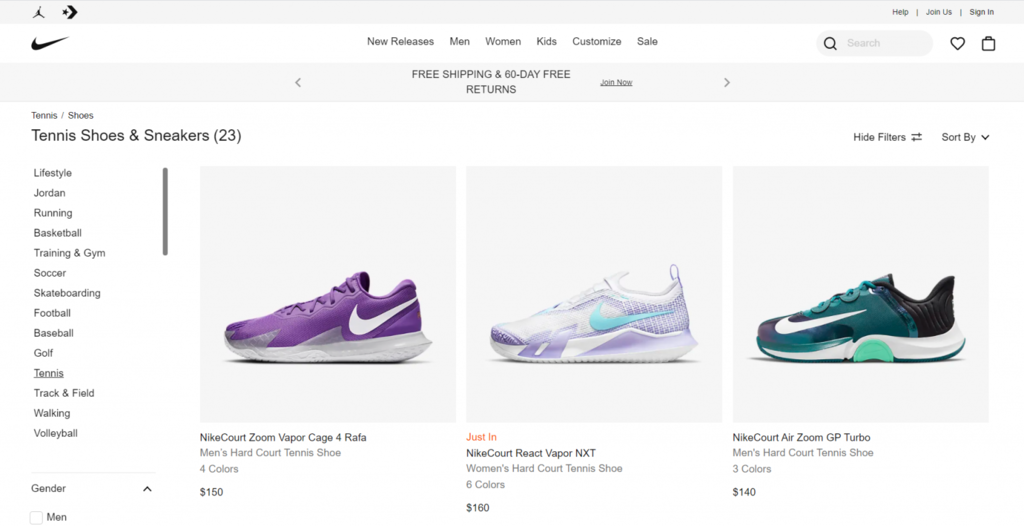This image is sourced from a sports clothing website with a clean, white background. The top features a light grey banner with a help menu and options to join or sign in. Below this is a white navigation bar offering clickable categories for new releases, men, women, kids, customized items, and sale items. Beneath the navigation bar is a search pill box accompanied by buttons for liking or adding items to the basket. The left-hand corner displays logos from brands like Nike and other sporting companies.

The current search query is for tennis shoes and sneakers, yielding 23 results. On the left-hand side, there are various filter options to narrow the search based on sports such as skateboarding, football, and baseball. The main section showcases three product images: a purple trainer on the left, a white and blue trainer in the middle, and a green trainer on the right.